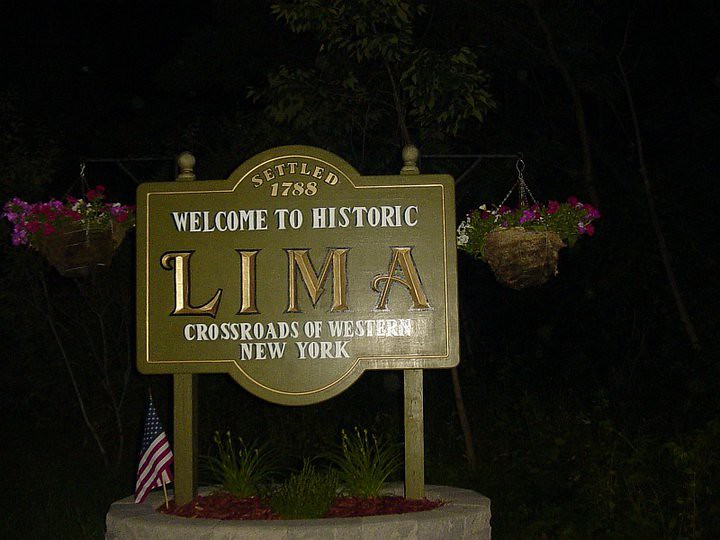This image features a prominent sign that reads "Welcome to Historic Lima," indicating the town's establishment in 1788 and lauding it as the "Crossroads of Western New York." The sign is centrally positioned in a circular stone structure reminiscent of a well, filled with soil and small patches of grass. Adding a patriotic touch, a small American flag protrudes next to the sign. Suspended on either side of the sign are flower pots, possibly containing some form of vegetation. The photograph appears to have been taken at night, as the surrounding area is shrouded in darkness, which highlights the illuminated sign and its details.